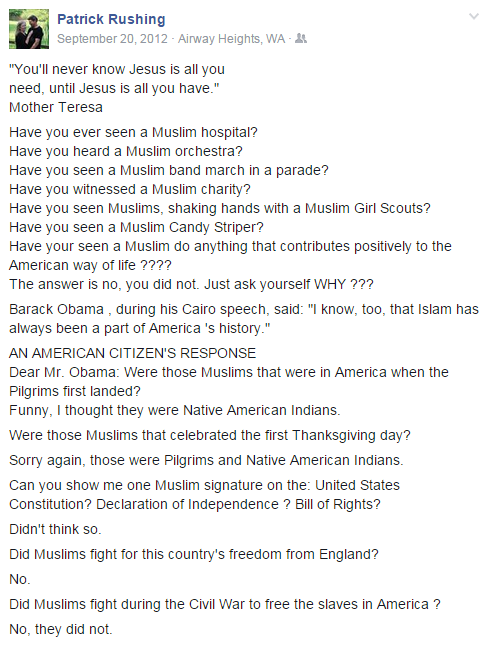On September 20th, 2012, Patrick Brushing from Airway Heights, Washington, shared a photo of a young couple looking at each other lovingly in a park, with the girl wrapping her arms around the guy. The post includes a quote from Mother Teresa: "You'll never know Jesus is all you need until Jesus is all you have."

Below the image, the post takes a controversial turn, posing a series of provocative questions: "Have you ever seen a Muslim hospital? Have you ever heard a Muslim orchestra? Have you ever seen a Muslim band march in a parade? Have you witnessed a Muslim charity? Have you seen Muslims shaking hands with Muslim Girl Scouts? Have you seen a Muslim candy striper? Have you seen a Muslim do anything that contributes positively to the American way of life?"

The post concludes these questions with an emphatic, "The answer is no, you did not. Just ask yourself why."

It transitions into a critique of Barack Obama's Cairo speech: "Barack Obama during his Cairo speech said, 'I know too that Islam has always been a part of America's history.' An American citizen's response, dear Mr. Obama, were those Muslims that were in America when the pilgrims first landed? Funny, I thought they were Native American Indians. Were those Muslims that celebrated the first Thanksgiving day? Sorry again, those were pilgrims and Native American Indians. Can you show me one Muslim signature on the United States Constitution, Declaration of Independence, Bill of Rights? Didn't think so. Did Muslims fight for this country's freedom from England? No. Did Muslims fight during the Civil War to free the slaves in America? No, they did not." The post ends abruptly at this point.